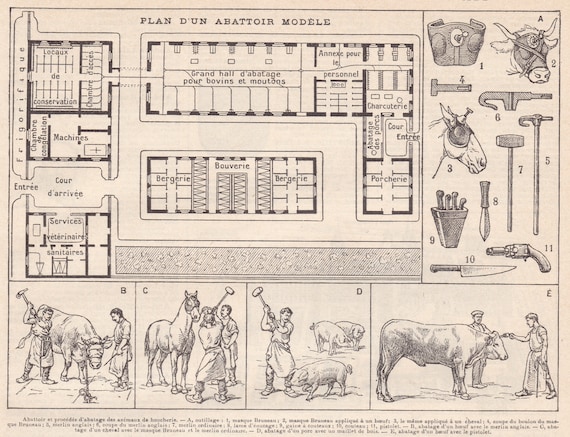This black-and-white diagram, labeled "Plan d'un Abattoir Modulé" (Plan for a Model Abattoir), presents a detailed floor plan of an abattoir designed for cows and sheep. The central building, marked as "Grand Hall d’Abattage pour Bouvines et Moutons" (Grand Hall for Cow and Sheep Slaughter), is surrounded by various annexes and specialized areas. To the left, annotations indicate facilities such as "le corps de conservation" (storage body), "chambre d’accès" (access room), "chambre congélation" (freezing room), "machines," and "cour d’arrivée" (arrival yard). Additional labels include "annexe pour le personnel" (staff annex), "charcuterie" (butchery), "porcherie" (pigsty), and "abattage des parcs" (slaughter parks). 

In the middle section, there are three labeled areas: "bergerie" (sheepfold) and "bouverie" (cattle stable), suggesting distinct zones for different types of livestock. The diagram also includes depictions of various equipment and methods used in animal slaughter. At the bottom are illustrations showing men using tools and devices on livestock: a sharp pick, hammers, a metal mask hit by a hammer, a bolt gun, and knives. One vivid image shows a man with a hammer raised over a pig, while another depicts a man about to use a gun on a cow's head. The entire layout is set against a gray background with black text, giving the diagram a stark and clinical appearance, evocative of early 20th or late 19th-century practices in animal husbandry.